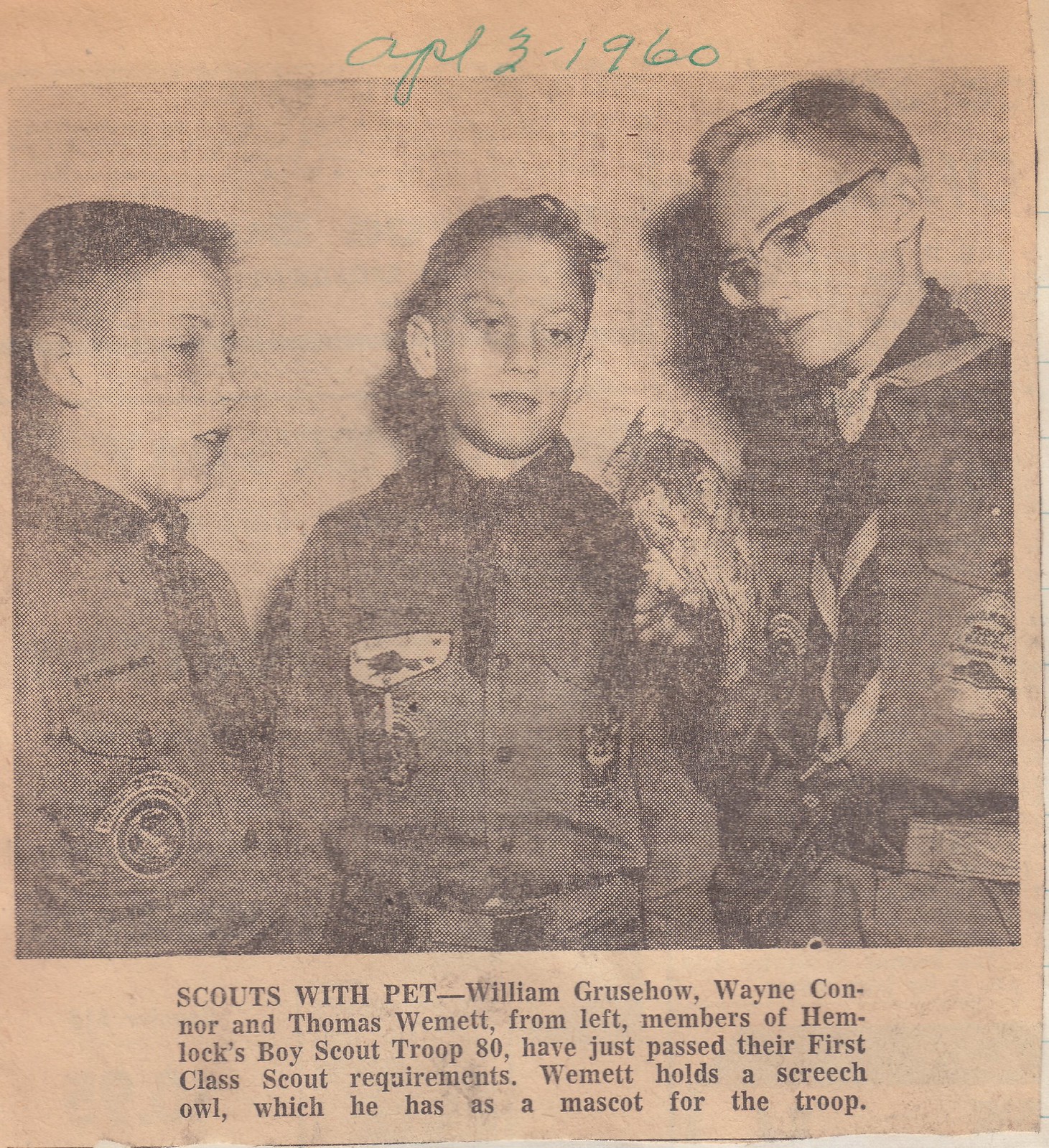The black-and-white image appears to be a cutout from a newspaper, marked at the top with "April 3, 1960" in green ink. It features three young boys dressed in Boy Scout uniforms, likely dark green given the context, each with short hair, except for the boy on the far right who is wearing glasses. From left to right, the boys are William Grusow, Wayne Connor, and Thomas Wemmett, members of Hemlock's Boy Scout Troop 80. Grusow faces to his right, showing just his right profile and the patch on his arm. Connor looks straight ahead and slightly down, revealing a patch and emblem on his right chest. Wemmett, on the far right, glances left and slightly down, holding a screech owl as a mascot for the troop in his right arm. The boys, all recently having passed their first-class scout requirements, seem to direct their gaze toward the owl. The caption below reads, "Scouts with pet," detailing their names and troop information, and confirming that Wemmett is holding the screech owl.